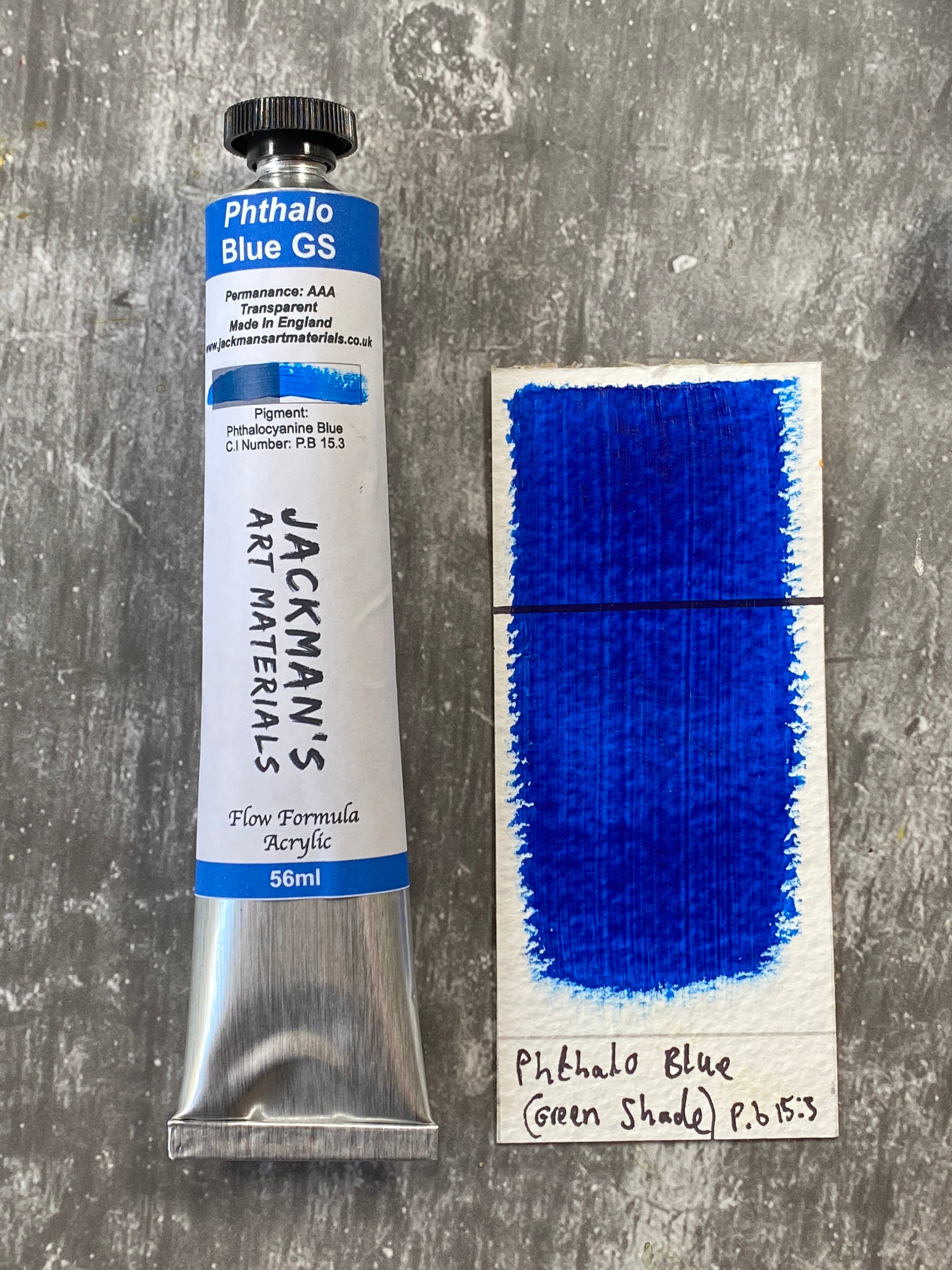This vertical rectangular image features a dark gray mottled background, possibly a table surface. On the left side of the image, there is a silver metallic tube of paint labeled "Jackman's Art Materials Flow Formula Acrylic, 56 milliliters." The tube has a black cap and a label in white and blue with additional black text. Prominently displayed on the tube is the paint color "Phthalo Blue, Green Shade (PB 15.3)" followed by "GS," indicating the green shade. Additional label details include the pigment information "Phthalocyanine Blue, PB 15.3," and notes on its permanence as "AAA" and its transparency. The tube also mentions being made in England with the accompanying website "www.jackmansartmaterials.co.uk."

To the right of the tube, there is a piece of white cardstock serving as a paint sample swatch, showcasing the color "Phthalo Blue, Green Shade (PB 15.3)." The blue color on the swatch is highlighted as a rough streak, matching the shade described on the tube. This setup allows viewers to see both the paint container and a visual representation of the paint color side by side.